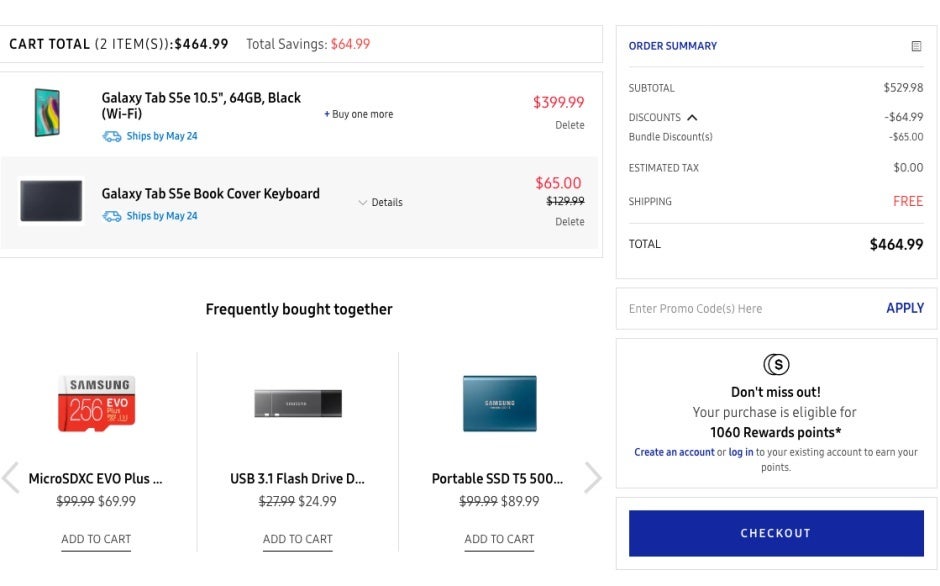**Detailed Caption:**

The image features an online shopping cart displayed on a clean, white background. On the left side of the screen, prominently written, is "Cart Total" indicating that there are two items in the cart totaling $464.99. Below this, in gray text, it mentions "Total Savings" with the amount $64.99 highlighted in red. 

The first item listed is the "Galaxy Tab S5e" which is described as a 10.5-inch, 64GB, black Wi-Fi model, priced at $399.99. It's noted that this item will ship by May 24th, with the shipping date highlighted in blue. Adjacent to this, there's a prompt suggesting to "buy one more." 

Below this, the second item listed is the "Galaxy Tab S5e Book Cover Keyboard," also shipping by May 24th. This item's price is marked down to $65 from its original price of $129.99, with an option to view "details." There's also a "delete" option next to this item.

Following this, there's a section for frequently bought together items. The first is a "Micro SDXC EVO Plus" reduced to $69.99 from $99.99, with an option to "Add to Cart." Next is a "USB Flash Drive" for $24.99, reduced from $27.99, followed by another "Add to Cart" option. Lastly, a "Portable SSD T5" is listed at $589.99, along with an "Add to Cart" button.

On the right upper corner of the image, the "Order Summary" section is visible. The subtotal is $529.98. After applying discounts of $64.99 and bundle discounts of $65, the total cost is adjusted. There's an "Estimated Tax" of zero and "Free" shipping written in red, leading to a final total of $464.99 written in black. Below this, there's an input field for entering a promo code, followed by a blue "Apply" button.

At the bottom, it mentions "Don't Miss Out! Your purchase is eligible for 1,060 reward points." It encourages users to "Create an Account" or "Log In" to an existing account to earn these points, with these options also highlighted in blue. At the very end, there is a blue banner with a "Check Out" button in white.